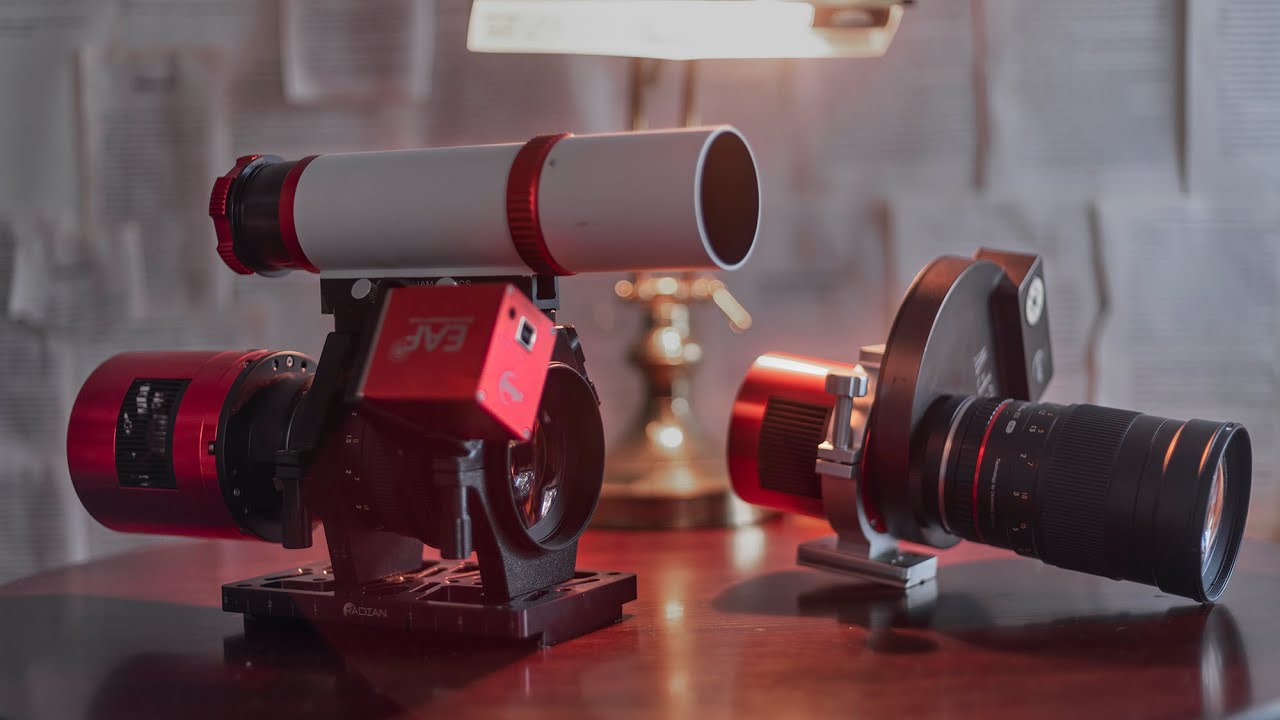This photograph captures a scene featuring two modified camera or telescope devices on a dark mahogany-toned wooden table, positioned just in front of a brass-based desk lamp with a white lampshade. In the background, a somewhat blurry but textured white wall can be seen, adding depth to the image. 

The object on the left is an improvised setup that includes a long-range camera lens attached to a metallic base with screws and clamps. It features a red cylinder and a red box, with additional components that appear to be parts of a telescope or camera strapped together in a homemade fashion. This device exhibits a mixture of black, red, and white elements, with red and black trim on a white pipe-like part and a lens at the far end.

To the right, there is another optical device that has a primary black lens and a large black base. This piece also incorporates a red metal section and is set up adjacent to the left object, both resting on the polished wooden surface. The combination of these elements, along with the muted, textured background and the elegant brass lamp, creates a visually intriguing scene of technological improvisation and creative assembly.